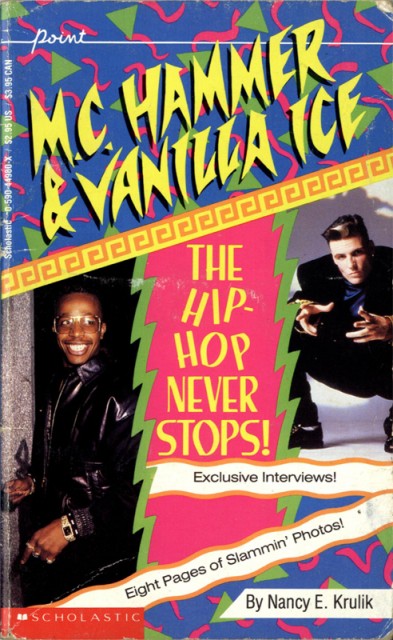The image is a vibrant, 90s-style book cover featuring prominent hip-hop icons MC Hammer and Vanilla Ice. At the top of the cover, the word "Point" is written in white. Directly below, in funky yellow font, it says "MC Hammer and Vanilla Ice," with each artist's picture positioned on the left and right respectively. The background is a dynamic mix of green triangles and pink swirls on a blue backdrop. A green border with red lightning bolt accents contains the phrase "The Hip Hop Never Stops" in bold yellow text. The cover also highlights, in white waves encircled by orange, "Exclusive Interviews" and "Eight pages of slammin' photos by Nancy E. Krulik." The bottom left corner features the Scholastic logo in red and white. The colorful and energetic design captures the essence of 90s hip-hop culture while promoting exclusive content within.